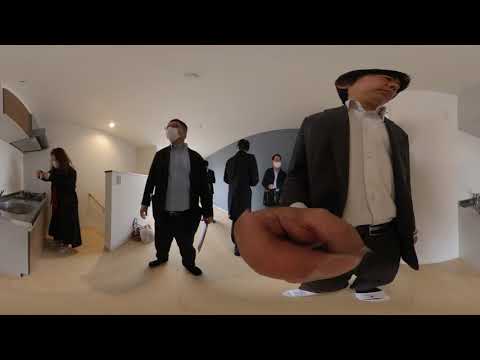In this image, a group of five people, all of whom appear to be Asian and are wearing masks, stand in a large, mostly empty room that appears to be part of a house or apartment. The setting features a tan floor and white walls, with a solid black border at the top and bottom of the image. The people are positioned centrally, some wearing business overcoats and white undershirts, while one man in the center stands out with a black overshirt and a blue undershirt, possibly holding a small object or a pole in his left hand. 

A woman dressed in a long black coat stands to the left over a kitchenette or sink, seemingly engaged in some activity. The room behind them is minimally furnished, with a large, white dome pillar prominently visible and a stairway descending to the left, illuminated by a light. The colors throughout the image include off-white, black, yellow, tan, blue, orange, and gray, creating a muted and clean aesthetic. Despite the indoor setting, it’s unclear what time of day the photo was taken as no natural light or windows are visible. The overall scene suggests a casual gathering, possibly aligned with current health guidelines given the masks.